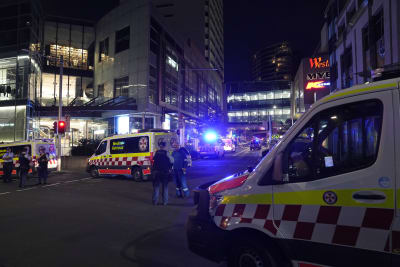In this nighttime outdoor city scene, the photograph captures a potentially serious incident involving multiple emergency vehicles. The image is rectangular, about two and a half inches wide by one and a half to two inches tall, and features a prominent white emergency van with yellow stripes and a red-and-white checkered pattern on its right-hand side. To the left are additional emergency vehicles, which appear blurred due to their distance. The scene is set at an intersection adorned with a red traffic light on the left and a green light towards the center.

Foreground details include several individuals in dark blue uniforms, likely emergency responders, with some wearing helmets and others crossing their arms, suggesting a state of readiness or assessment. The backdrop is dominated by towering skyscrapers with illuminated windows and signage, including a partially legible sign reading "West... Ace." The ambient light primarily emanates from the buildings and streetlights, accentuating the urban landscape.

The scene hints at an accident or crime, suggested by the concentration of emergency personnel and the nature of the emergency vehicles, which stylistically indicate the setting might not be the U.S.—potentially a European city. Despite the hustle and presence of responders, the specific cause of the assembly remains unclear, underpinning a sense of urgency and potential peril.